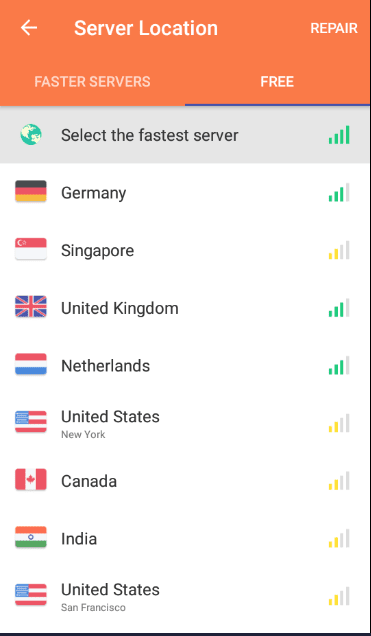Screenshot of a VPN Mobile App Server Selection Screen:

At the top of the screenshot, there's a header that reads "Server Location," flanked by a back arrow on the left for navigation and a "Repair" dialogue option on the far right. Directly below, two selection buttons are displayed: "Faster Servers" and "Free," with the "Free" option currently highlighted. 

Beneath these options, there's an image of a globe in white and green, with an accompanying label that reads "Select the Fastest Server," featuring an icon indicating a strong connection with five bars. Following this are a list of server locations alongside their signal strength:

- Germany with four bars,
- Singapore with two bars,
- United Kingdom with three bars,
- Netherlands with three bars,
- United States (New York) with two bars,
- Canada with two bars,
- India with two bars,
- United States (San Francisco) with two bars.

This screen is particularly notable for displaying two separate server locations within the United States, one in New York and the other in San Francisco.